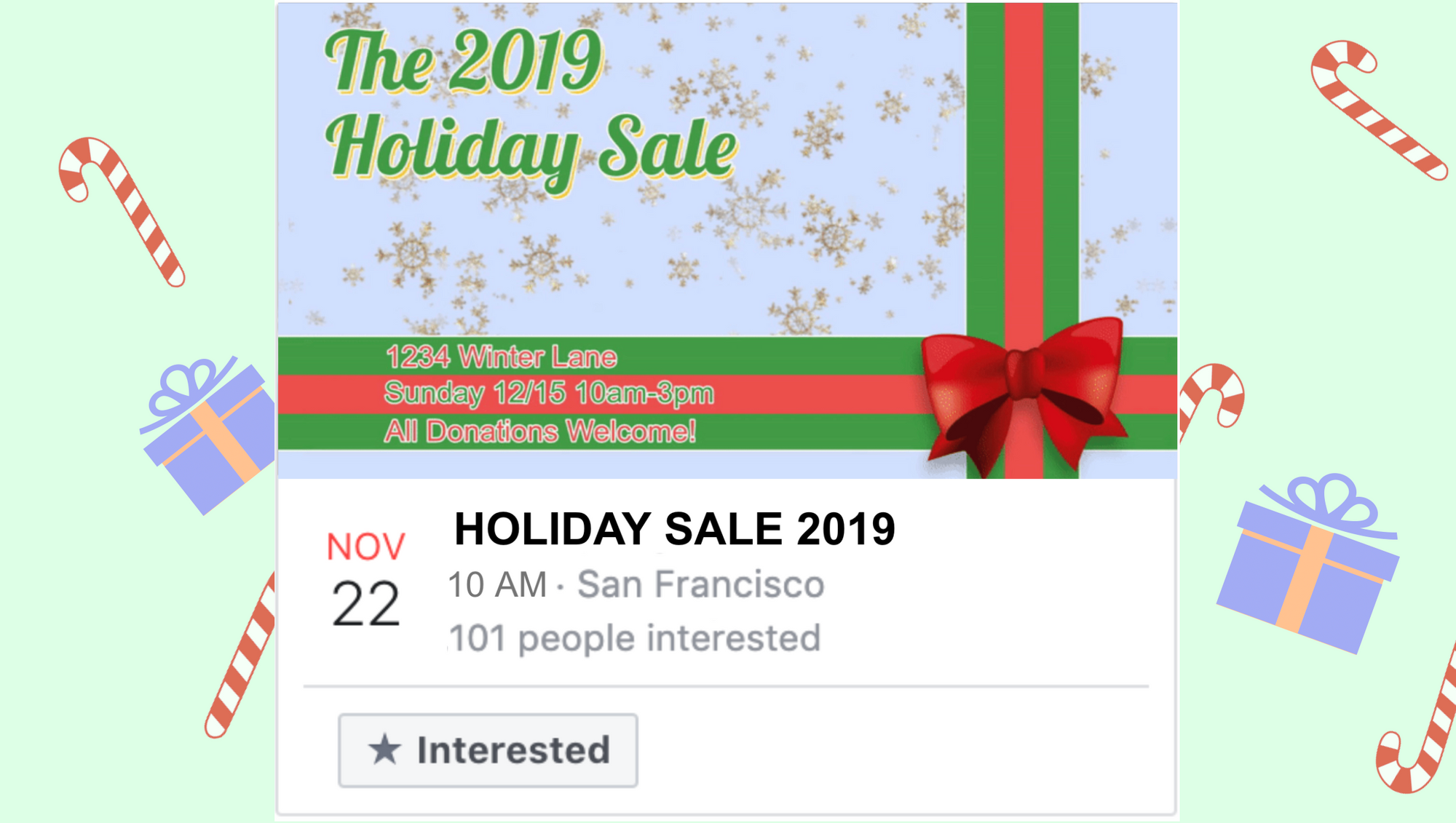**Descriptive Caption:**

The image is a detailed screenshot of a website showcasing a holiday event. The sides of the webpage are bordered with light green, pistachio-colored banners adorned with whimsical drawings of candy canes and presents. 

In the center of the page, a festive graphic is featured against a blue background with gold snowflakes. At the top of this section, green text announces "The 2019 Holiday Sale." Below this, green and red ribbons cascade down both sides and meet at the bottom in a red bow, creating a cheerful holiday motif. 

Further down, critical event details are displayed: "One Two Three Four Winter Lane, Sunday 12/15, 10 a.m. to 3 p.m.," all in red text, except for the event date and time, which are in green. A message encouraging donations is also highlighted in red.

Adjacent to this, a white background box features the abbreviation "NOV" in red print, with "22" in black print beneath it. This is followed by bold, capitalized text that reads "HOLIDAY SALE 2019," and below it, the event time and location, "10 a.m. San Francisco" along with "101 people interested."

Additionally, there is an interactive element: a button labeled "Interested" with a gray star next to it, designed in gray text with a capital "I."